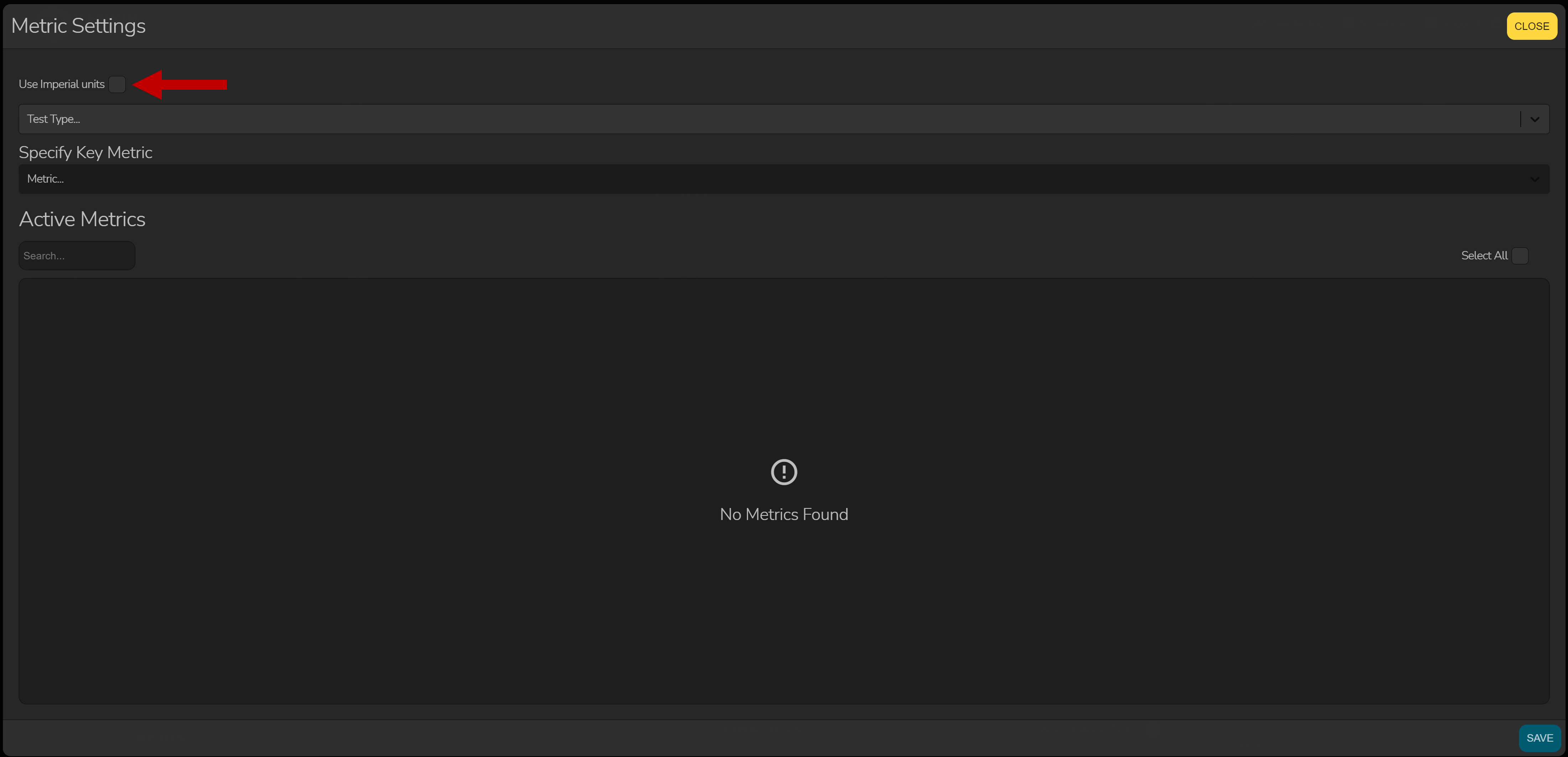The image is a screenshot of a webpage's settings area with a dark color theme. The background is predominantly black and gray. At the top of the image, there is a solid black rectangle that spans the entire width of the screen. On the upper left corner of this rectangle, "Metric Settings" is displayed in white font. On the upper right corner, there's a small yellow rectangle with the word "Close" in black font, indicating a clickable button.

Below this top section, there's a darker black rectangle. A red arrow has been added to the image, pointing to a small checkbox which users can click to select an option called "Use Imperial Units," written in gray font.

Further down, there's a lighter gray drop-down menu with the placeholder text "Test Type..." in white font. Underneath this, the text "Specify Key Metric" appears in white font.

Proceeding further down, another small black rectangle is visible, containing some white text that is not legible in the screenshot. Below this, the section titled "Active Metrics" is present. Under the "Active Metrics" section, there is a search field where users can type in their queries. To the far right of this search field, "Select All" is written in white font, with an accompanying checkbox next to it.